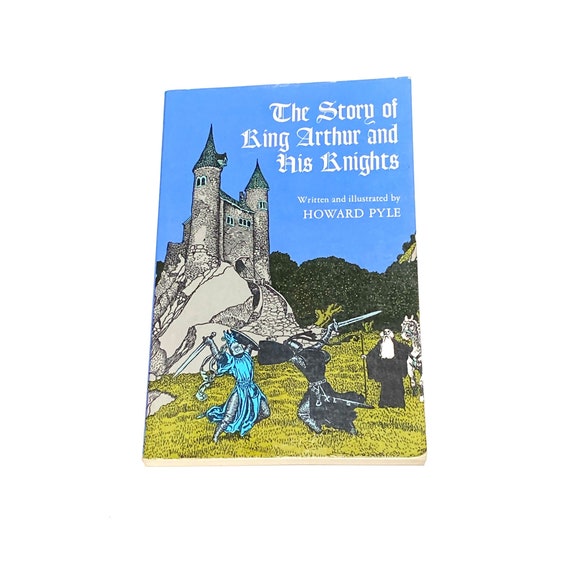The image is a detailed photograph of the cover of a book titled "The Story of King Arthur and His Knights," written and illustrated by Howard Pyle. The cover illustration captures a dynamic battle scene set in a bright, clear day on a grassy field. Two characters are prominently depicted in the foreground engaged in a sword fight: one garbed in a light blue outfit and the other in black. To the right, a figure that resembles a religious or wise man with a long white beard stands beside a horse, observing the duel. In the distance, a majestic gray castle with green roofs sits perched on a rock formation, surrounded by a stone walkway, green trees, and rolling hills under a blue sky. The text of the title and the author's credit appear at the top in white letters, set against the backdrop of this vivid and colorful medieval scene. The colors used in the cover range from various shades of blue and green to teal, off-white, and gray, giving it a rich and lively appearance. The complete image of the book's cover is visible, including a slight view of the lower edges of the pages due to the book being tipped back slightly.